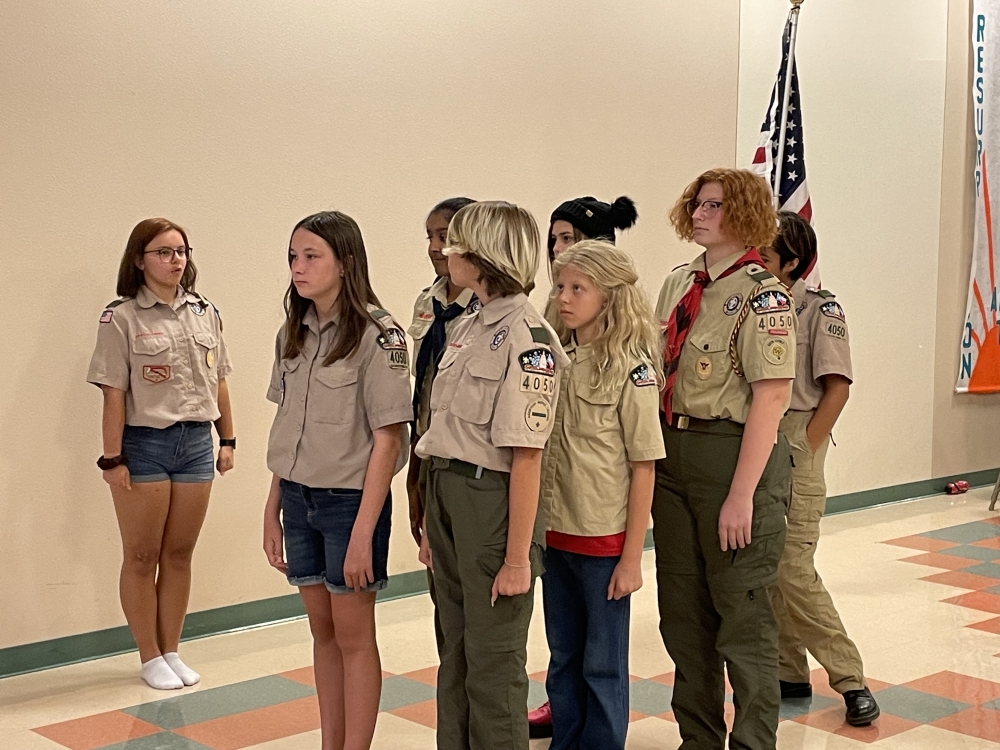The photograph depicts a group of young Cub Scouts, identifiable by their beige collared shirts adorned with various patches and badges, including a visible troop number "4050." The Scouts, comprising both boys and girls, approximately seven in total, are standing in two orderly lines in what appears to be a school setting. The scene is framed by beige walls with a green baseboard and a floor tiled in green, red, and beige. An American flag on a pole is positioned in the background to the right. One Scout, possibly a leader, stands near the left side of the image, facing the group and appearing to give commands, while the others mostly look straight ahead or towards the leader.